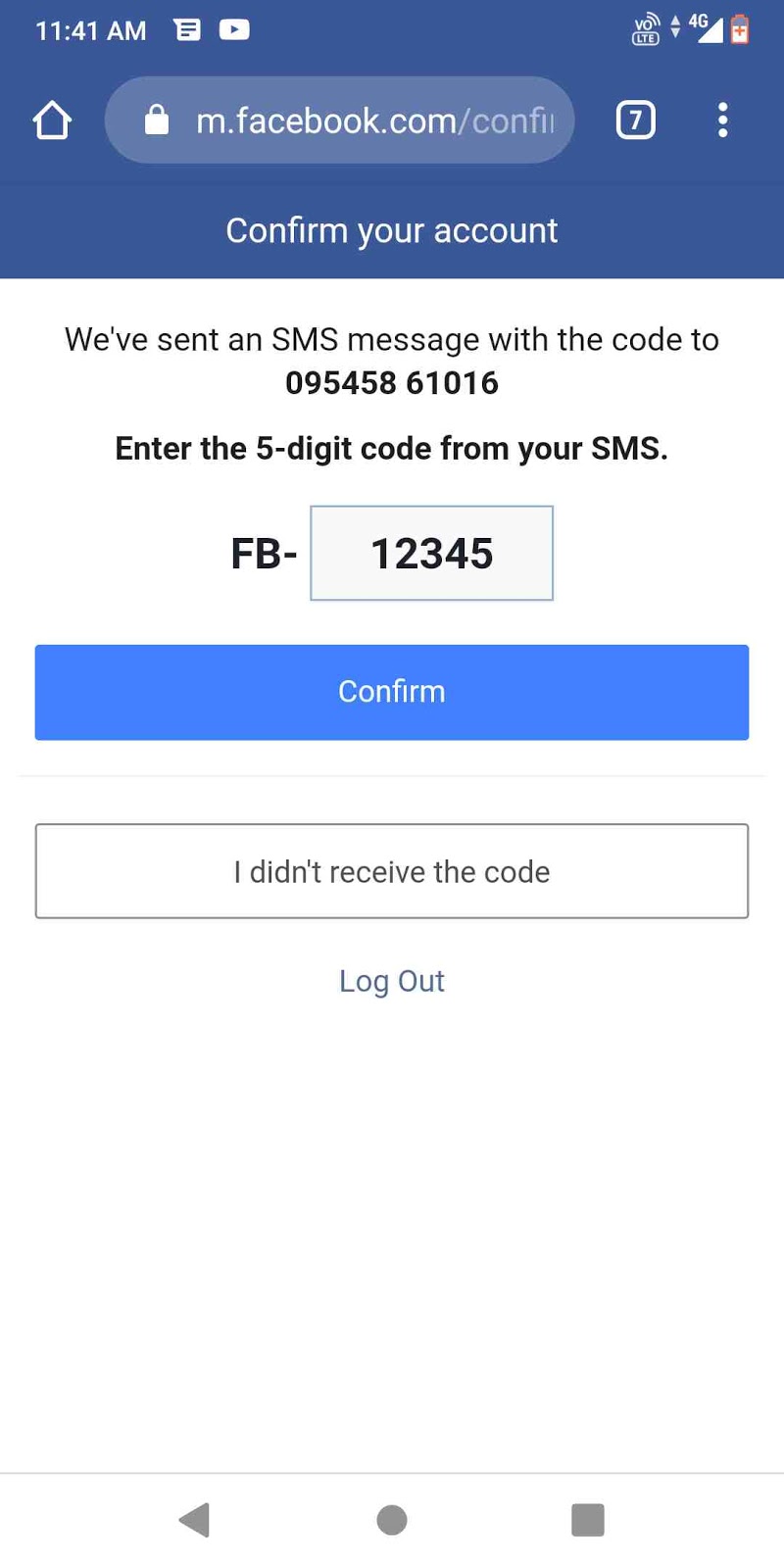The image depicts a section of a Facebook screen displayed on a cell phone. A range of icons at the top confirm this: the timestamp reads 11:41 AM on the top left, accompanied by icons such as a messaging icon and a YouTube icon. Towards the right, typical phone indicators are visible, showing a connection bar and a battery icon indicating approximately 60% charge.

Beneath these indicators is the URL "m.facebook.com". Adjacent to the left of the URL is a home page icon, while the right side displays a tab number, "7", followed by three vertical white dots indicating additional options.

The main content area below these icons contains a prompt to confirm the user's account. The text reads: "We've sent an SMS message with the code to 09545861016. Enter the five-digit code from your SMS." Below this message, 'FB' is shown beside a gray input box containing the placeholder "12345". The background in this section, as with the rest of the image, is white.

Further down, there is a light blue rectangular button with the text "Confirm" centered within it. Below this, a gray rectangular button states "I didn't receive the code," and below that is a "Log out" option.

At the very bottom of the screen, there are three additional phone navigation icons: a sideways triangle on the left, a circle in the middle, and a gray square on the right. These icons signify navigation functions and complete the depicted section of the cell phone screen.